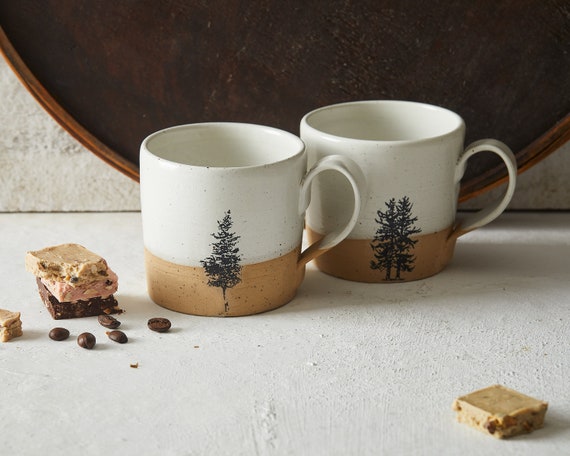The image displays two coffee mugs on a white, textured surface. Each mug is designed with a predominantly white upper section and a light brown base, including white handles with brown detailing. Both mugs feature an evergreen tree illustration on the front, with the left mug partially obscured by the one on the right, giving the appearance that the trees are aligned to form a cohesive design. To the left of these mugs, there is a small dessert item comprising two stacked squares—the top one is a lighter brown, possibly peanut butter or fudge, with a darker brown square beneath it. Surrounding this dessert piece are scattered coffee beans. Another similar light brown square of the dessert is located in the lower right corner. In the background, a circular wooden tray is propped up against a light-colored, rough-textured wall.